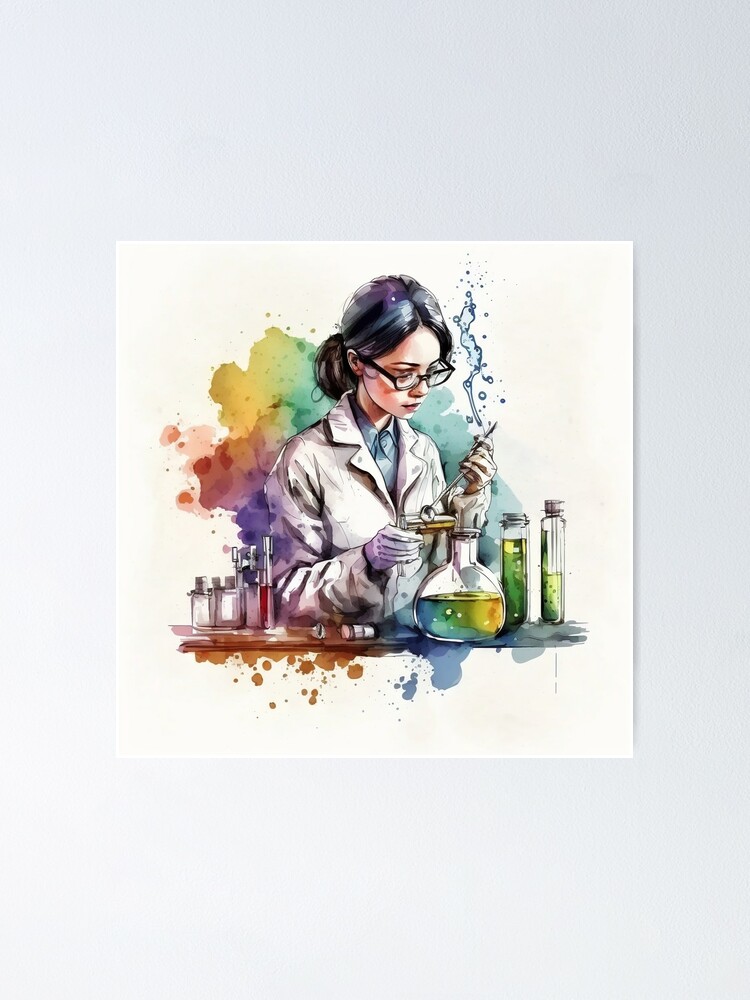This is a detailed digital rendering of a young female chemist, showcasing her in a laboratory setting. She appears to be either Caucasian or possibly Asian and is depicted with long, dark hair tied back into a ponytail. She wears black-rimmed glasses, a white lab coat, and purple gloves, over a light blue dress shirt. In her hand, she holds an ambiguous instrument, likely a pipette, from which blue smoke emanates.

In front of her, a variety of scientific glassware is arranged on a brown countertop. Notably, there's a prominent, large bottle featuring a vibrant gradient of orange, yellow, green, and blue liquid. Adjacent to it are two tall beakers containing green liquid, one nearly full and the other filled slightly less than halfway. Further to her right (the viewer's left), several small bottles are visible: one contains a red substance, while the others appear either empty or filled with clear or gray material.

The background is mostly blank white with an artistic addition of multicolored paint splotches in shades of red, yellow, green, blue, and purple, enhancing the vibrancy of the scene. Additionally, there's a multicolored smoke effect directly behind her, adding to the dynamic and creative visual appeal of the image. She is shown carefully observing and possibly conducting an experiment, epitomizing the diligence and focus of a dedicated scientist.